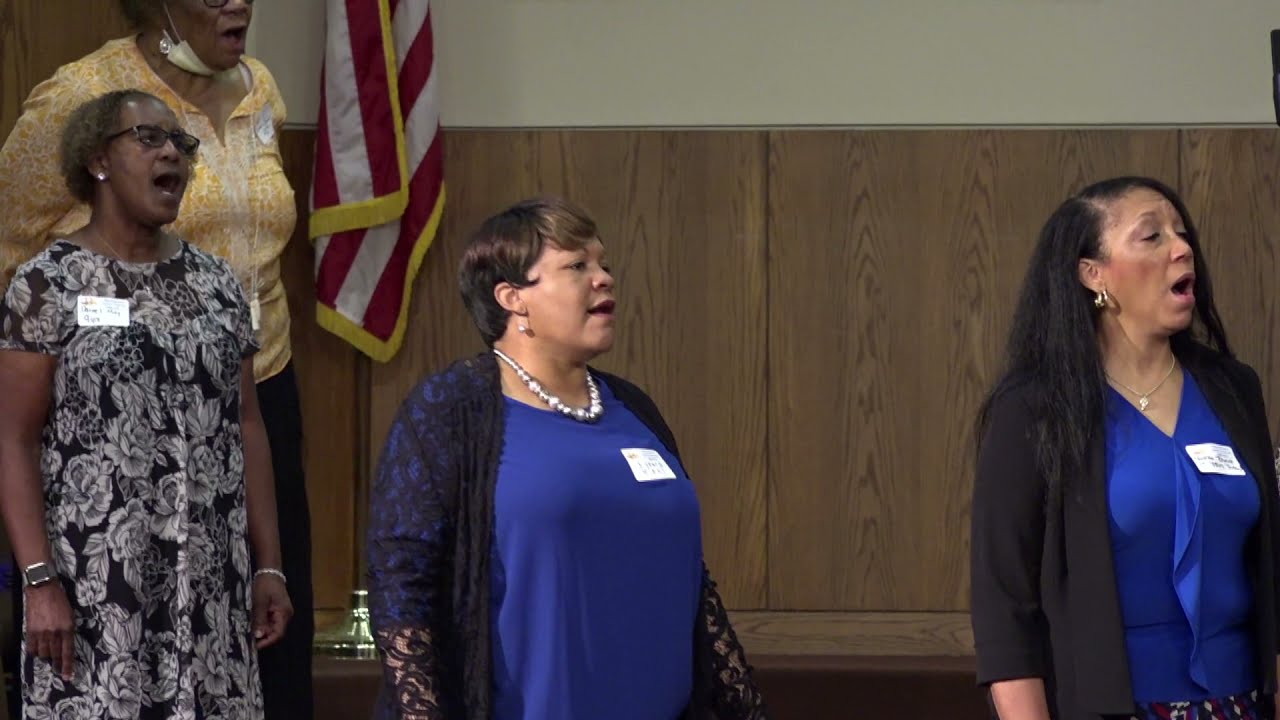In this vivid screenshot from a video, we observe a group of four African American women, part of a choir, captured mid-song. They are visually communicating a harmonious performance, spaced apart which might suggest COVID-19 precautions. The lady positioned towards the back dons a yellow blouse and a mask that is lowered to below her chin, emphasizing the pandemic undertone. In the foreground, three women wear name tags and distinctive outfits: one in a dark dress, two in blue tops with layered clothing. Specifically, one woman adorns a black and white floral dress paired with glasses, a second sports a blue shirt and black cardigan accentuated with a white necklace and earrings, and the third, distinguishable by long black hair, has a blue blouse with a black sweater jacket. Their animated expressions and open mouths convey the vibrancy of their singing.

The backdrop features classic brown paneling juxtaposed with white wainscoting and a greenish or beige wall. An American flag stands prominently to the left, bordered in gold, adding a touch of patriotism to the setting which suggests a possible church or community hall.